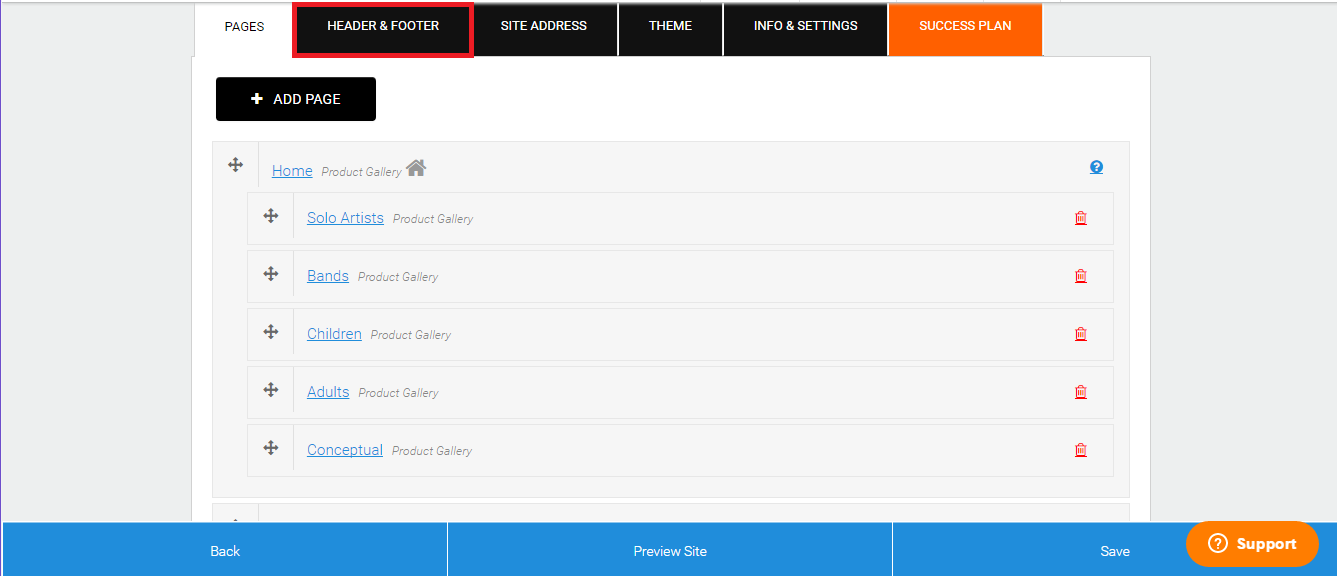The image appears to depict a music-related interface, possibly a settings or selection page, characterized by various organizing elements and selectable options:

In the upper section, there is a prominent blue rectangle with a blue band at the bottom, alongside an orange "Support" button. Below, the interface consists of multiple horizontal rectangles, each with black backgrounds and white text. Key sections within these rectangles include "Site Address," "Theme Info," "Settings," and "Success Plan," the latter of which is highlighted in orange. Notably, "Header and Footer" is outlined in red, drawing attention to this area.

Additionally, there is an "Add Page" option followed by navigational headings such as "Home" and "Product Gallery." Below these sections, various categories are listed, such as "Solo Artists," "Bands," "Children," "Adults," and other conceptual buttons, all of which can be selected. The top category, "Blue," is currently highlighted, while the other categories feature small red icons, indicating some form of display or action. The overall arrangement and color coding suggest a well-structured menu, aimed at organizing content related to music themes.